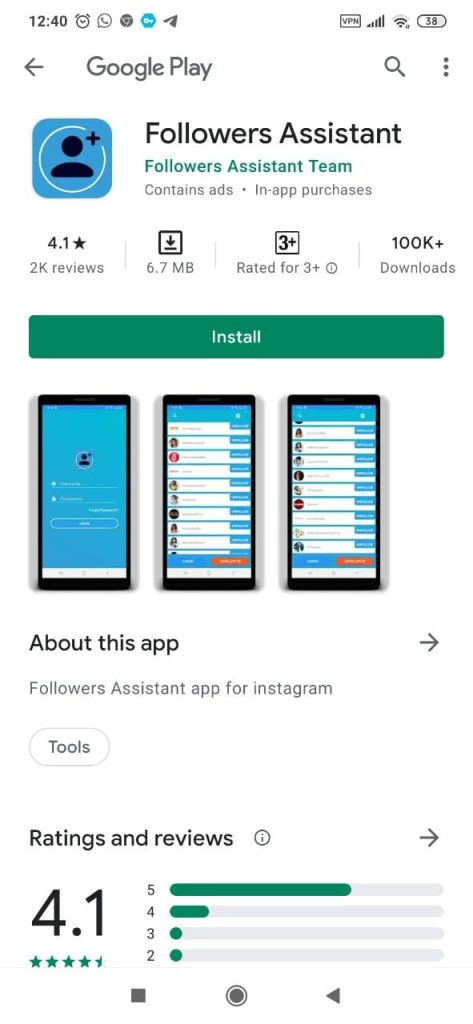**Detailed Caption of the App Store Screenshot:**

This image is a screenshot of an application page from a mobile phone app store, displayed on a white background. At the very top left corner, a dark grey text reads "12:40." To the right of this, there are multiple icons, followed by some negative space. On the far right, there are four icons also arranged horizontally.

Beneath this header, another dark grey arrow points leftwards, accompanied by the text "Google Play," also in dark grey. To the right, amid some more negative space, there is a dark grey magnifying glass icon followed by three vertically stacked dark grey dots.

In the next section, on the left, there is a blue square with rounded corners, containing a generic black profile picture icon. A black plus symbol appears at the top right of this profile icon, and a white circle outline fills the rest of the blue square around the profile picture icon. 

To the right of this blue square, on the white background, bold black text reads "Followers Assistant." Below this, smaller blue text states "FOLLOWERS ASSISTANT TEAM," and under this, light grey text mentions "Contains ads," followed by a centered grey dot, and finally "In-app purchases" to the right.

Further below, several sections are divided by thin light grey vertical lines. The first section on the left features black text stating "4.1" with a black star icon to its right. Underneath this, light grey text reads "2K reviews." The adjacent section to the right displays a black download icon, with light grey text underneath indicating "6.7 MB." The following section states "3+" inside a black box, with light grey text below reading "Rated for 3+," accompanied by a light grey eye icon encircled in grey. The final section to the right shows "100K+" in black text, with "Downloads" underneath in light grey.

Directly beneath these sections, a green button with white text reads "Install." Below this button, three images of a mobile phone screen are displayed. The leftmost screen is predominantly blue, while the two screens to the right show vertical stacks of white rectangles with blue buttons on the right and profile icons on the left.

At the bottom of the screenshot, "About this app" is written in black text on the white background, with a dark grey arrow pointing to the right following the text.

The screenshot ends at this point, with additional content likely continuing further below.